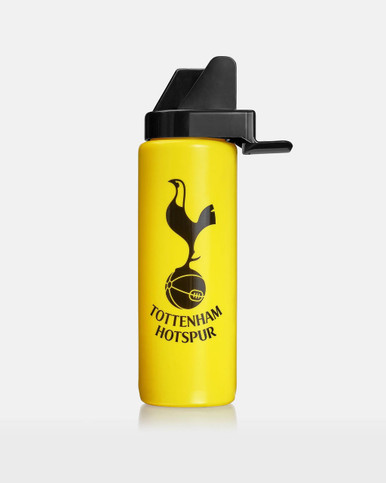The image features a yellow cylindrical plastic bottle set against an almost white background with its light reflection visible beneath it. The bottle's black plastic cap includes a small, flat piece on the right side that protrudes slightly and may serve as a mouth spout or drinking point. The top of the cap is circular, with a section extending to the right and flattening out. The front of the bottle displays a black graphic of a bird standing on a spherical object, resembling a basketball or medicine ball, with the text "Tottenham Hotspur" arched upward beneath it.